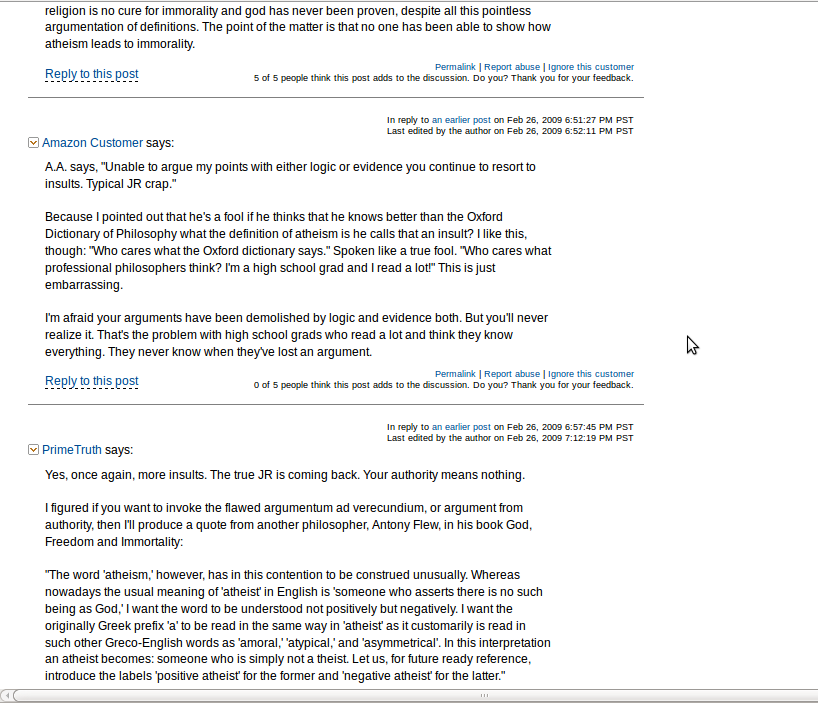A cropped screenshot captures a contentious exchange in a comment section, framed against a stark white background. The topmost comment is partially visible, but the primary focus is on the second comment, positioned near the top center of the image. The comment is attributed to "Amazon Customer," who laments their inability to argue their points with logic or evidence, citing frequent resort to insults as "typical JR crap." The customer is critiquing another individual for dismissing the Oxford Dictionary of Philosophy's definition of atheism, branding the dismissive attitude as foolish. They mockingly summarize the opposing view as disregarding the importance of professional philosophers, substituting it with self-confidence derived from being a high school graduate who reads extensively. The customer concludes that this overconfidence is ultimately embarrassing and asserts that the arguments have been decisively refuted by logic and evidence, although they doubt this will be recognized by the opponent.

Visible at the bottom left of the comment is an option to "reply to this post," presented as a hyperlink. To the right, there are additional options to "permalink," "report it," and "ignore this customer," highlighting standard features of a comment moderation system. Additional context is provided by a following comment listed under the name "prime truth," suggesting that the screenshot is from a comment-enabled platform, mirroring Amazon's user interface rather than an actual review section.